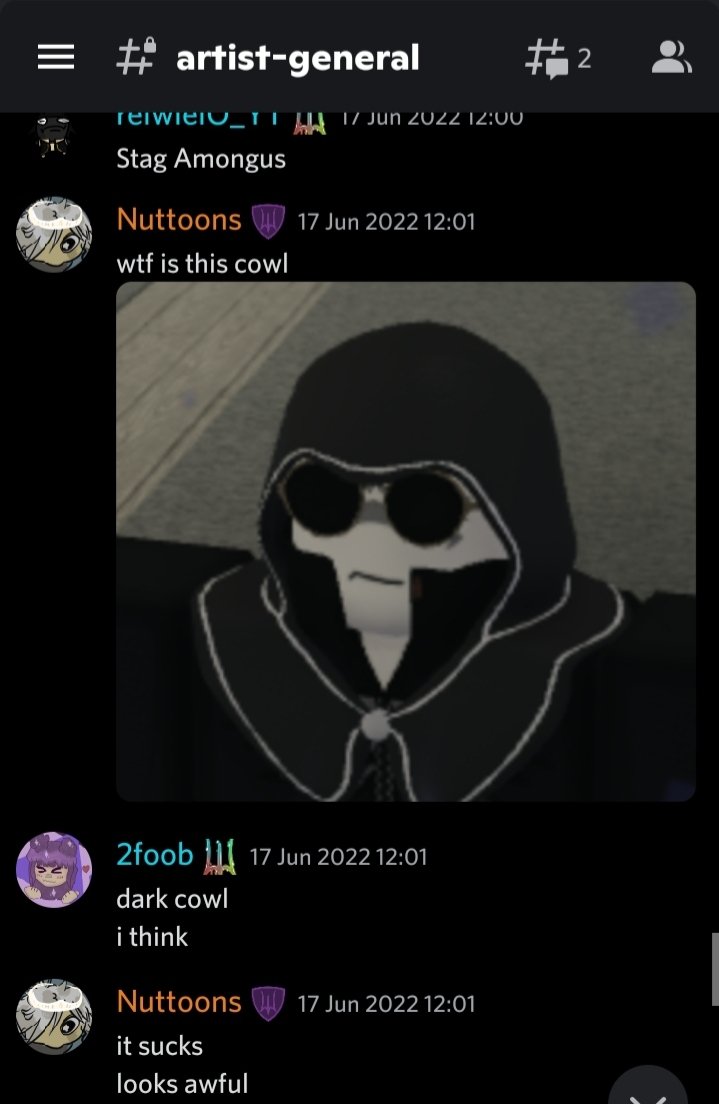The image is a screenshot from a phone. In the top left corner, there is an icon with three horizontal lines stacked vertically, indicating a menu. Next to it, the text "Artist-General" is displayed. Below this heading, there is a timestamp reading "17 June 2022 at 12:00," along with a partially visible message starting with "stag among us." 

Following this, at 12:01, a user named "No Tunes" comments "WTF is this cow," referring to an illustration. The illustration itself depicts a person standing against a gray background, wearing a black hood that covers their head, along with round black glasses. The hood's collar extends up to the person's upper cheeks.

The next message, also timestamped at 12:01, is from a user named "Foob," who states, "dark cow I think." Below, another comment from "No Tunes" at the same time simply says, "it sucks looks awful."